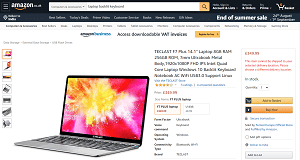Screenshot of an Amazon webpage displaying a selected laptop product. At the top-left corner, the familiar Amazon logo is prominently featured. The central portion of the header is dominated by a search field, flanked on the right by three small, indistinct options and a shopping cart icon. Unfortunately, due to the image's small size, the precise details of these options are unclear.

Beneath the main header lies a blue navigation banner, typical of Amazon's interface, populated with menu options that are similarly difficult to discern due to small font size in the screenshot.

Directly below the banner, the laptop product page is visible. The main visual is a high-resolution image of an open laptop. On the left side of this section, additional thumbnail images of the laptop are arranged vertically, allowing for alternative views upon clicking.

To the immediate right of the main image, a concise summary of the laptop is provided. This section includes user reviews, the product price, and key laptop specifications. Further right, there is an additional information section highlighted with red font details, which remain unreadable at this zoom level. 

Finally, accompanied by a yellow and an orange button, this far-right section likely offers purchasing options, such as "Add to Cart" and "Buy Now."